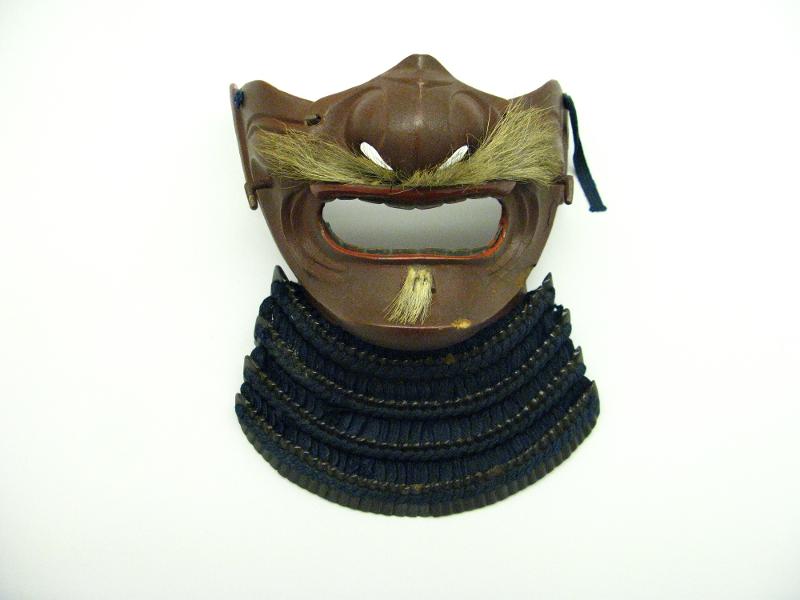This image showcases the bottom half of a theatrical mask, likely inspired by Japanese Kabuki or Noh theater traditions. The mask, primarily light brown in color, is detailed with an intricately designed, slightly comical appearance. It features a prominent gold mustache and a small goatee which appears to be made of fake blonde hair. The nose area is well-defined, while the mouth is an open oval, seemingly designed to allow the wearer's real mouth to be visible through it.

Noticeably, the mask is highlighted with a subtle dark orange rim around the lip area. The top of the mask appears broken or irregular, adding to its distinctive character. Enhancing its theatrical flair, the mask includes a decorative collar below, consisting of four layered bands, which may be made of rope or cloth, presumably to cover the wearer’s neck. Set against a stark white background, the intricate details and striking features of this mask are brought clearly into focus.